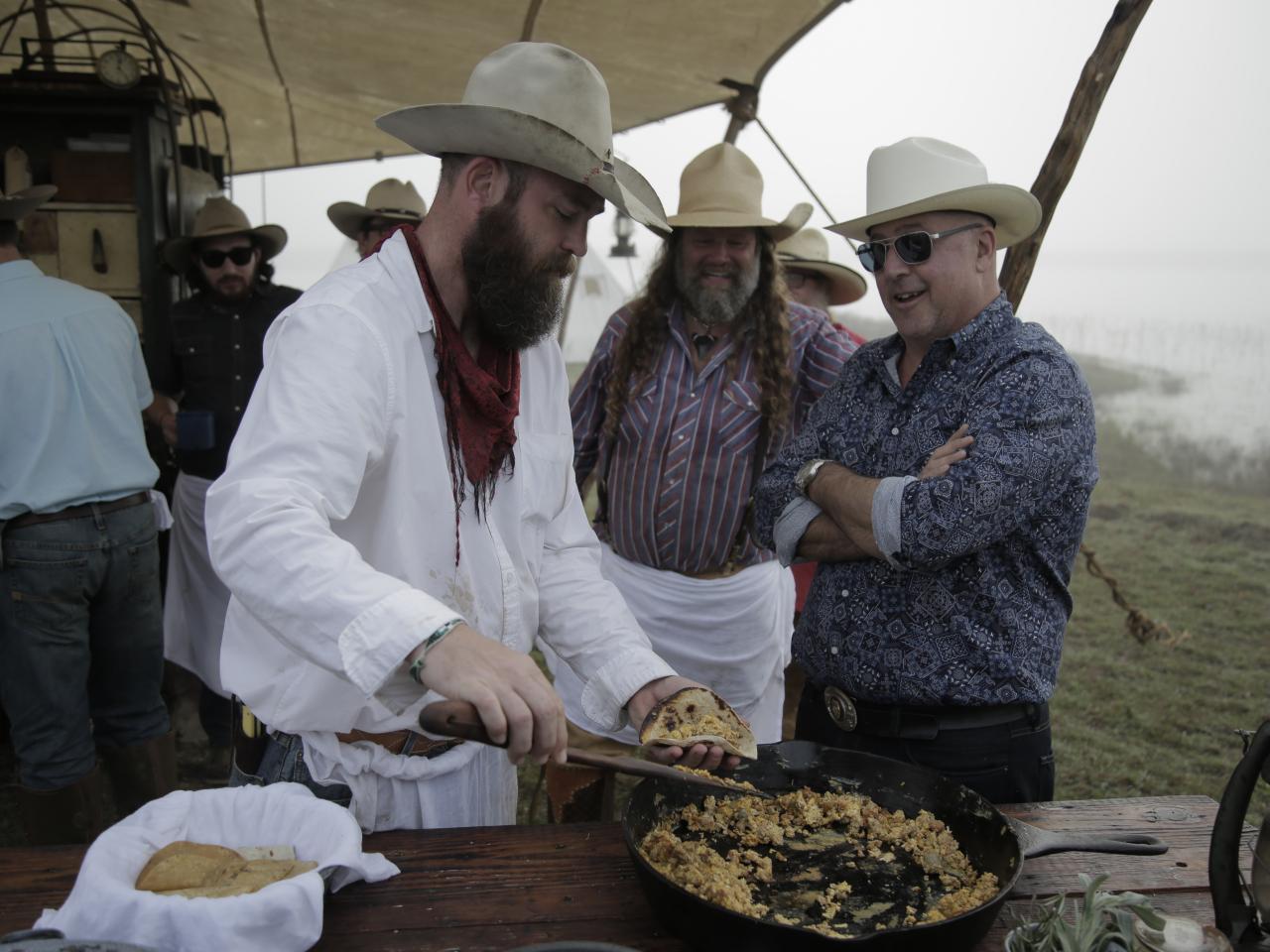In this color photograph, a group of men are gathered around a modern-day chuck wagon, reminiscent of those used by cowboys in the 1800s. The setting is outdoors on an overcast, gray day, by a marshy area or body of water. A tent overhead provides some cover. 

At the forefront, a man with a tan cowboy hat, a long brown beard, and a white long-sleeved shirt with a red bandana is seen scooping chopped-up chicken, or perhaps hash or eggs, from a large black cast-iron skillet into a tortilla using a wooden spoon. He has a white towel tied around his waist. To his left stands another man wearing a striped button-up shirt, a light-hued cowboy hat, and an apron, with long hair draped over his shoulder. On their right, another man leans casually with crossed arms, sporting a light-colored cowboy hat, sunglasses, a paisley shirt, and a belt buckle with dark pants.

In the background, other figures can be faintly made out, also wearing cowboy hats, contributing to the historical ambiance of the scene. The wooden countertop in front is strewn with cooking supplies, including a bowl containing additional tortillas.